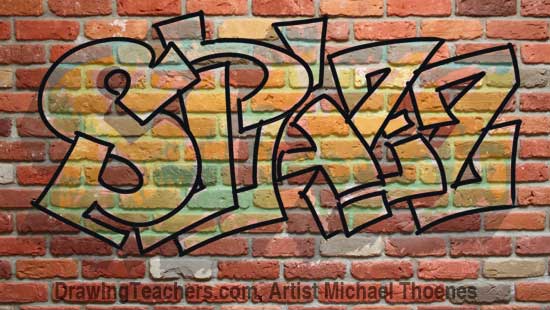This digitally created image depicts a red brick wall with a mixture of horizontal red bricks and occasional white or gray bricks. Along the bottom of the image, text reads "DrawingTeachers.com, Artist Michael Thoenes (T-H-O-E-N-E-S)." Spanning from one end of the wall to the other is a piece of graffiti art that spells out "SPAZZ" (or possibly SPLAZZ, though it's difficult to distinguish). The graffiti appears in stylized, boxy bubble letters with a light yellow-greenish tint and a black outline. The letters are semi-transparent, allowing the brick background to show through, giving them a clear, smoky appearance. Shadows beneath the letters add depth and enhance the realistic feel of the digitally drawn artwork. The overall shape of the image is horizontal, mimicking the format of a banner or website advertisement.